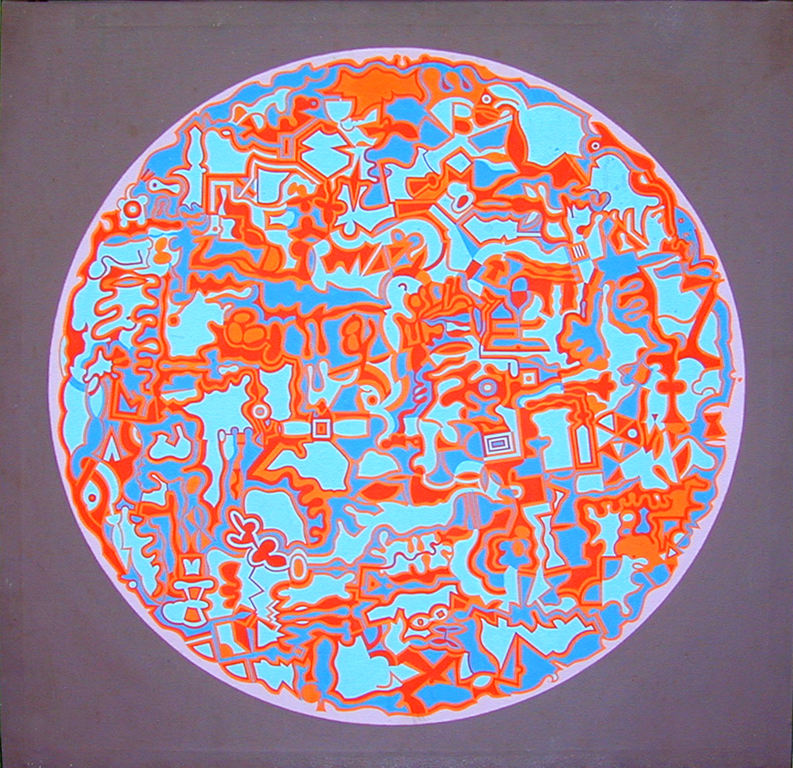The image is a detailed photograph of colorful artwork, displayed in a centralized, round format on a flat, gray fabric surface characterized by visible creases, especially noticeable along the edges and the wrinkled top right corner. The artwork itself features a light pink border and an array of random shapes with no discernible pattern, heavily utilizing hues of light blue, dark blue, light orange, and orange. The orange often appears as borders or lines, while the light blue dominates larger shapes, and the dark blue is seen in standalone forms.

The composition presents a colorful, multicolored art piece centralized in the image. There are no textual elements associated with the artwork. The round illustration is set within a square frame, giving the impression of an organized yet abstract piece. This artwork, evocative of a silicon wafer, is a color illustration attributed to an Australian artist and is part of the Computer History Museum's collection. The variety of shapes within the circle includes squares with highlighted blue centers and puzzle piece-like forms, all adding to the visual multiplicity of the piece.